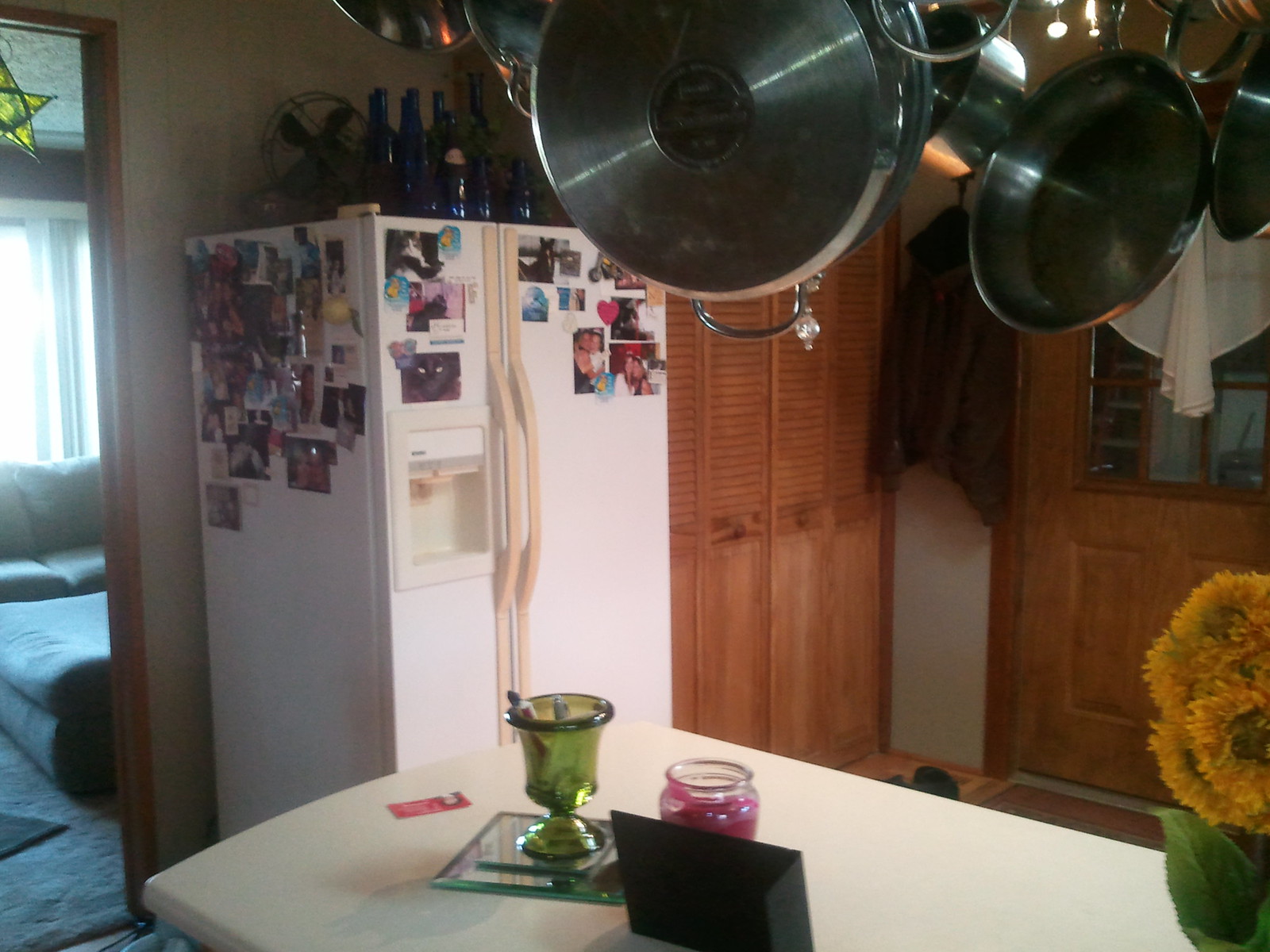The photo showcases a cozy kitchen area with various detailed elements. In the top right corner, several pots are hanging from a suspended rack. Beneath them, a white table holds a small green container filled with markers or pens and a pink glass candle beside it. A black picture frame faces away, adding a touch of elegance. In the lower right corner, vibrant green leaves with yellow flowers brighten the scene. 

On the left side, a white side-by-side refrigerator features an ice and water dispenser and is adorned with numerous photos, covering both doors and the upper area. Atop the refrigerator sit tall blue bottles and the black blades of a floor fan. 

To the left of the refrigerator, an open doorway leads to another room. A star decoration dangles from the ceiling above a brown rug. Further into the room, a plush, soft blue couch invites comfort and relaxation.